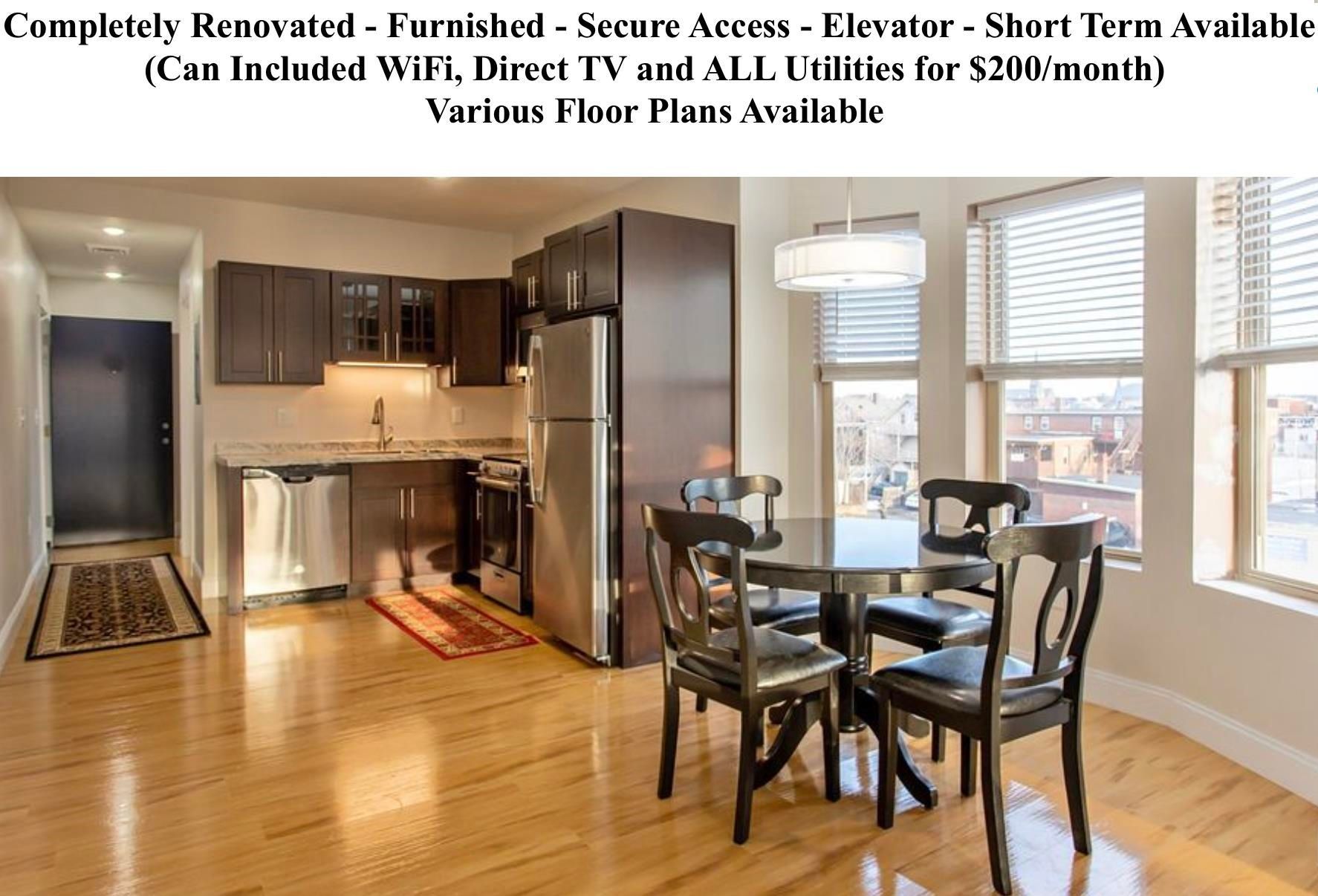This image appears to be part of an advertisement showcasing a fully renovated and furnished apartment. At the top of the image, text in black on a white background highlights the key features: "Completely renovated, furnished, secure access, elevator, short-term available." It also mentions optional inclusions in parentheses: "Can include Wi-Fi, DirecTV, and all utilities for $200 a month." Followed by the additional note, "Various floor plans available."

Below this textual information, a photograph offers a glimpse into the apartment's interior. On the left side, a door opens into a hallway adorned with a rug, leading into a well-equipped kitchen. The kitchen features a fridge, freezer, oven, stovetop, sink, and dishwasher, complemented by overhead cabinets for storage. More towards the right, there's an open space with a circular dining table accompanied by four chairs. Along the wall adjacent to the dining table, three windows with blinds pulled halfway up allow natural light to fill the room, giving it a warm and inviting ambiance.